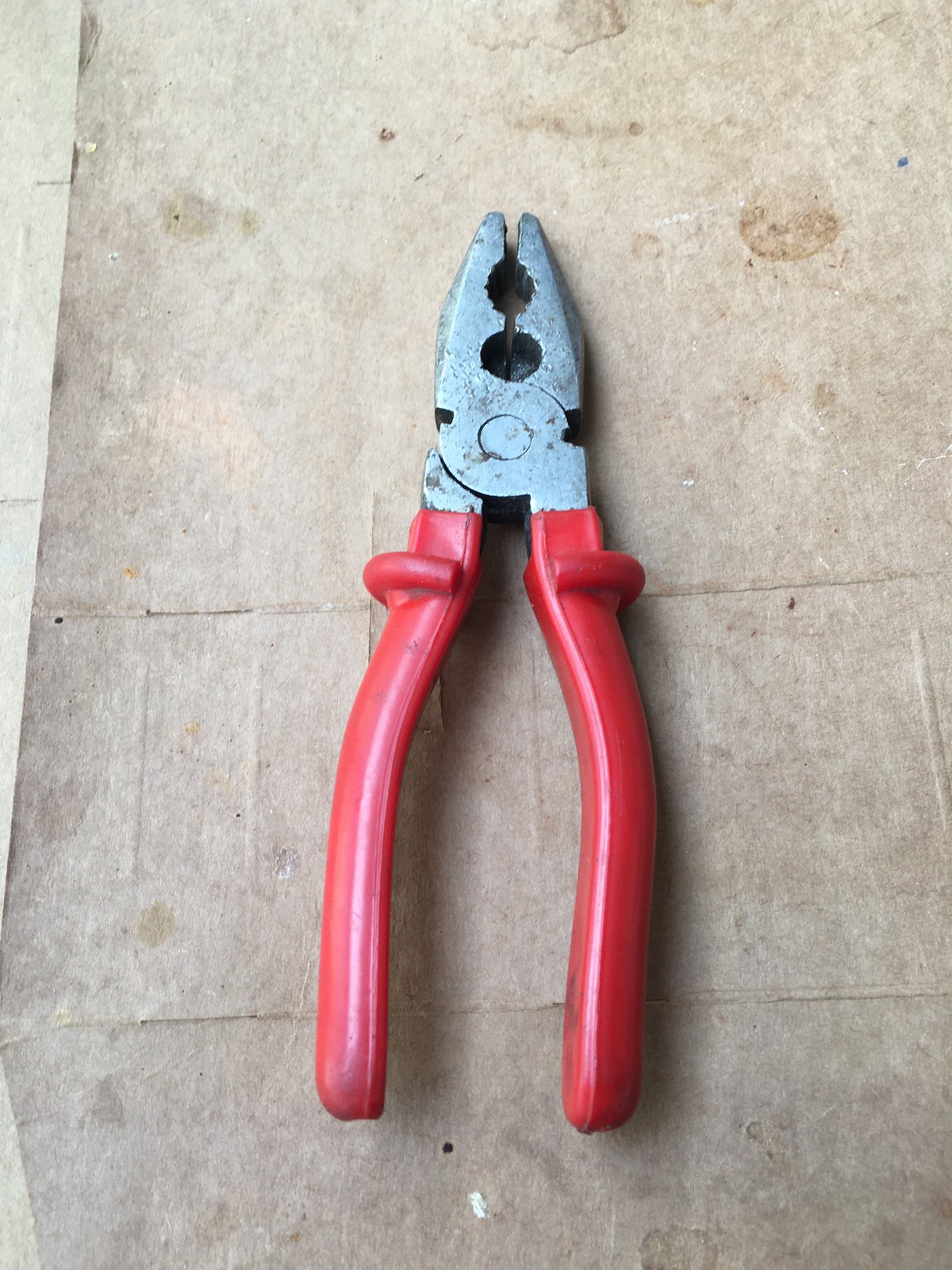A color photograph captures a vintage-looking pair of pliers laying flat on a dirty, stained ground that appears to be a greyish-brown surface, potentially with some grassy texture. The pliers, positioned with the handles towards the bottom and the metal jaws at the top, are centrally placed in the image. The long handles are coated in red, possibly rubber, and feature a textured detail near the top. The metal part of the pliers is silver but shows signs of wear with some chips and blackened areas, especially towards the bottom sides. The pliers also include a wire stripper, with the hinge secured by a central bolt, and culminate in a slightly pointed, somewhat flat tip. The surface beneath the pliers is marked with stains, spots, and possibly a couple of intersecting cracks, adding to the overall aged and rugged appearance of the scene. Towards the left corner, a lighter grey area borders the image, further complementing the weathered backdrop.